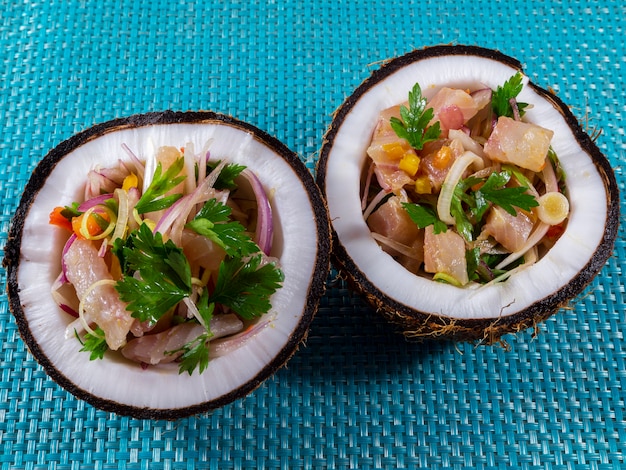The image showcases a vibrant and detailed food presentation featuring two equal halves of a coconut, split horizontally, and positioned on a blue, knitted or wicker-style mat. The hollowed-out coconut shells serve as natural bowls filled with a bright, colorful salad. This salad appears to include chopped vegetables such as red onion, tomato, and carrots, along with leafy greens like cilantro. There are also cubes of fish or crab meat, giving it a seafood twist. The different textures and colors of the ingredients create a visually appetizing display, with the coconut shells casting noticeable shadows under the light. The overall effect is a beautiful and enticing display of a fresh, tropical-inspired mixed salad using the coconut as unique serving vessels.